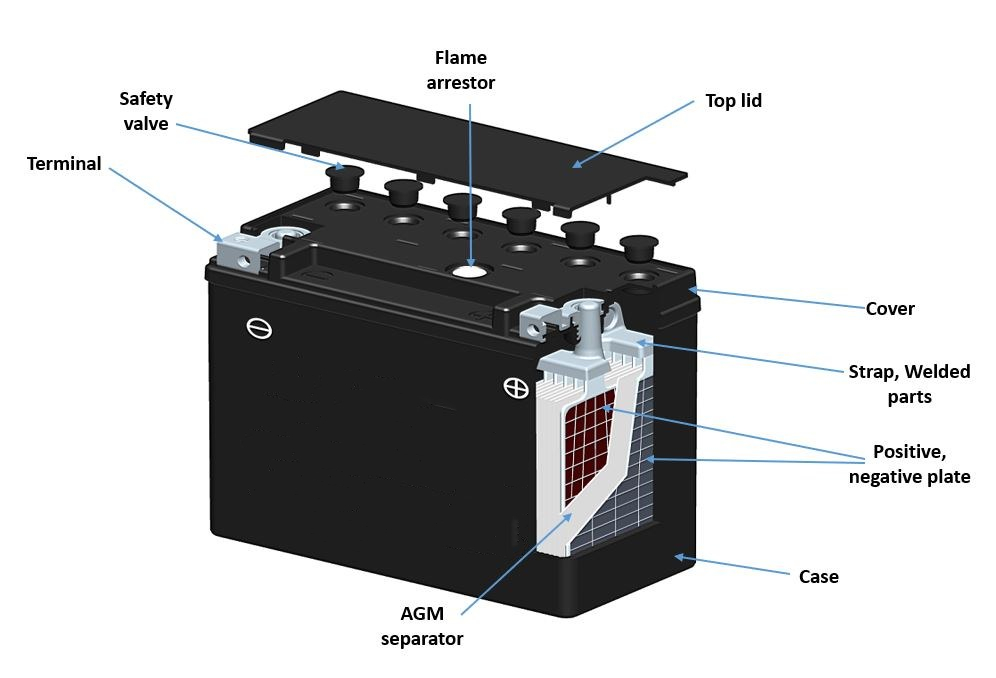The image is a detailed diagram illustrating the components of a battery. The battery, approximately the size of a car battery, is housed in a black case with sections of the exterior opened up to reveal the internal components. Various parts of the battery are labeled with arrows in light blue. Key elements identified include the terminal, safety valve, flame arrestor, top lid, cover, strap, welded parts, positive and negative plates, case, and AGM separator. The diagram uses colors such as gray, white, light gray, red, and light blue for clarity, and emphasizes the different metal alloys used in the construction of the battery. The top lid is depicted as detached to provide a better view of the inside.